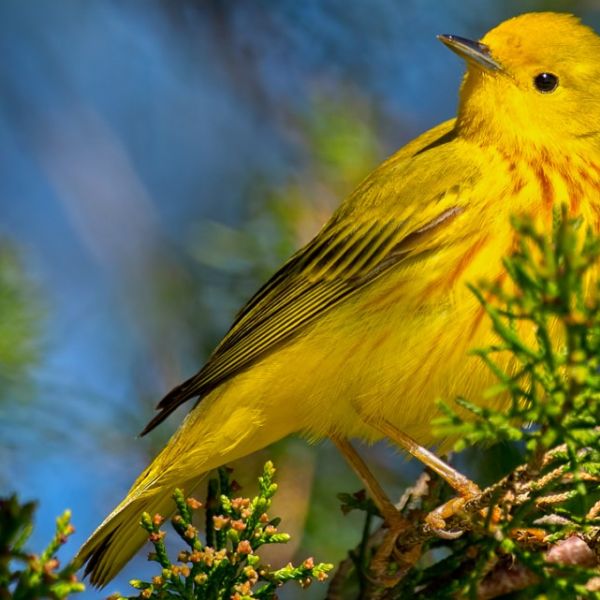In this close-up photograph, we see a remarkably beautiful yellow bird, likely a member of the finch family. Positioned sideways, the bird's chest faces east while its tail points west, and its head is turned upward. The bird boasts a striking yellow head and chest, complemented by intricate black striping on its upper wings. Its black eye and beak add a captivating contrast to its vibrant plumage. The bird's golden-colored legs are wrapped securely around a branch, conveying a sense of delicate determination. Surrounding the branch is lush greenery, while the background is artistically blurred, featuring hints of blue sky and green trees in the upper left-hand corner, adding depth and atmosphere to the scene.